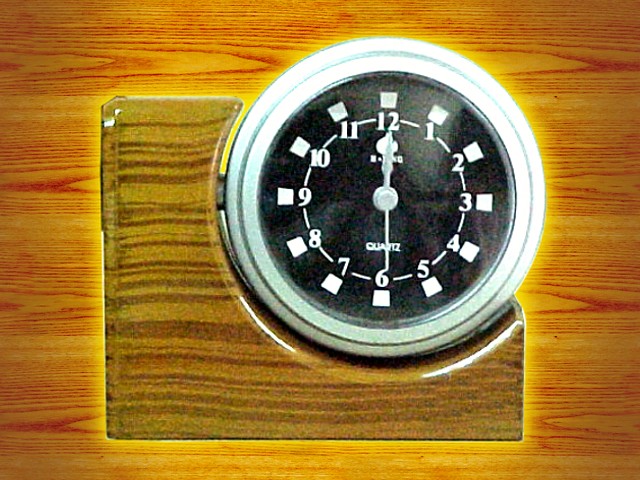This photograph depicts a distinctive wooden clock. The clock is encased in a yellow wood with a striking red horizontal grain. At the center of this wooden base sits a round clock bordered with a sleek silver edge. The clock face is black, featuring bold white numbers and whitish-colored hands. Each number from 1 to 12 is accompanied by a small square marker. The word "Quartz" is also printed on the clock face. The clock is elegantly displayed on a wooden stand, which consists of a square piece of wood with a semi-circular cutout, creating a moon-shaped arc that supports and cradles the round clock.